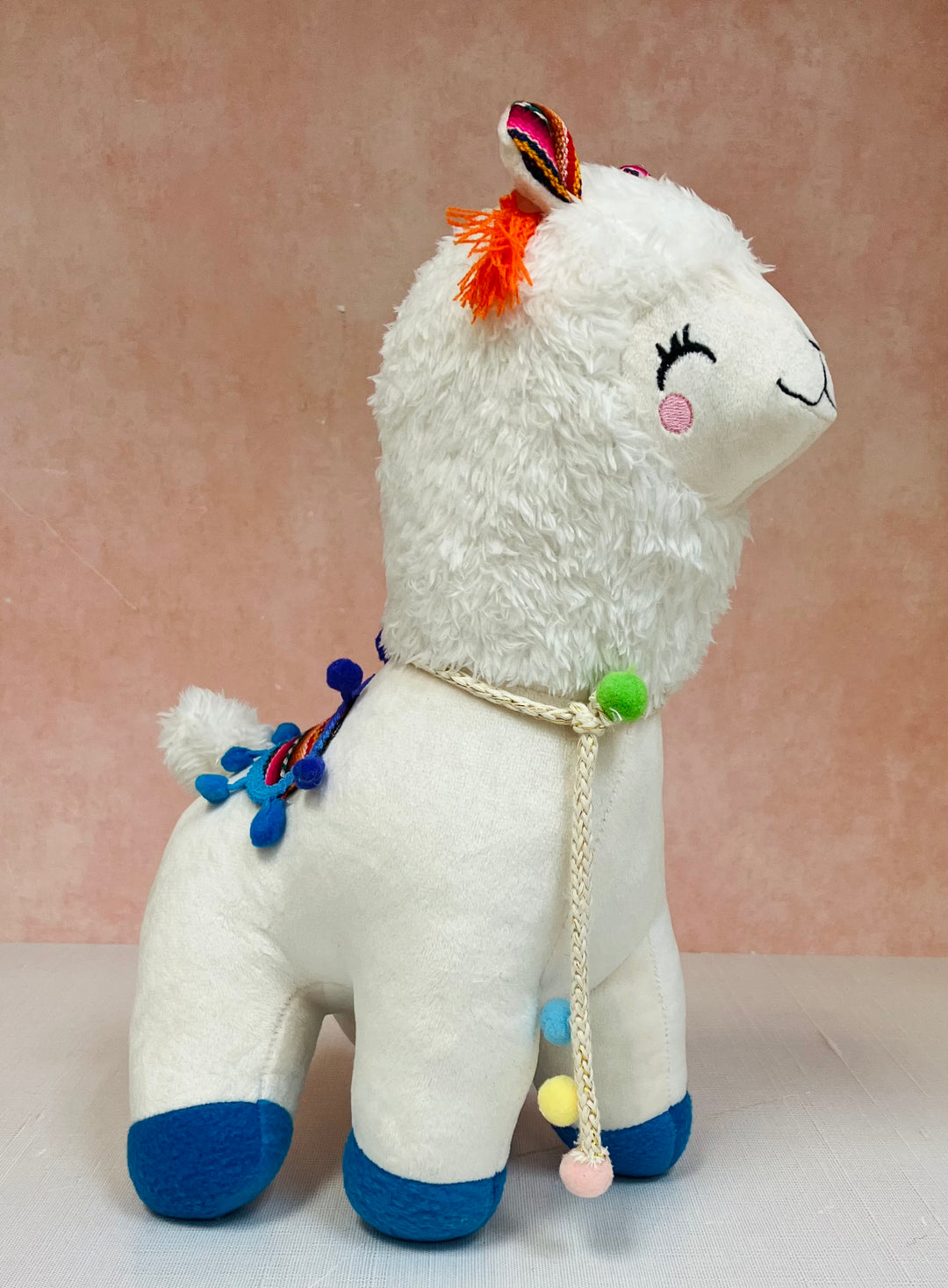This color photograph in portrait orientation features a plush toy that appears to be a llama. The llama is positioned centrally, standing on all fours on a white surface, facing the top right of the image. The background behind it is a pinkish-peach color.

The llama has a smooth, white body adorned with a colorful blanket on its back, which is blue with blue felt balls outlining it. Its feet are covered in blue fabric. The head of the llama boasts fluffy, white fur with a tuft of orange string-like hair at the top. 

The llama has closed eyes, depicted as black lines with eyelashes above them, and a pink circle on its right cheek, visible just below the right eye. The ears are upright, featuring a colorful inner lining with an Aztec print that includes purple, orange, and black on the front, and white on the back.

Around its neck, the llama wears a white rope that hangs down in front, with a green ball at the top, and smaller blue, yellow, and pink balls at the bottom. The overall style of the photograph is a blend of photographic realism and representationalism, capturing intricate details of the stuffed animal’s features and accessories.